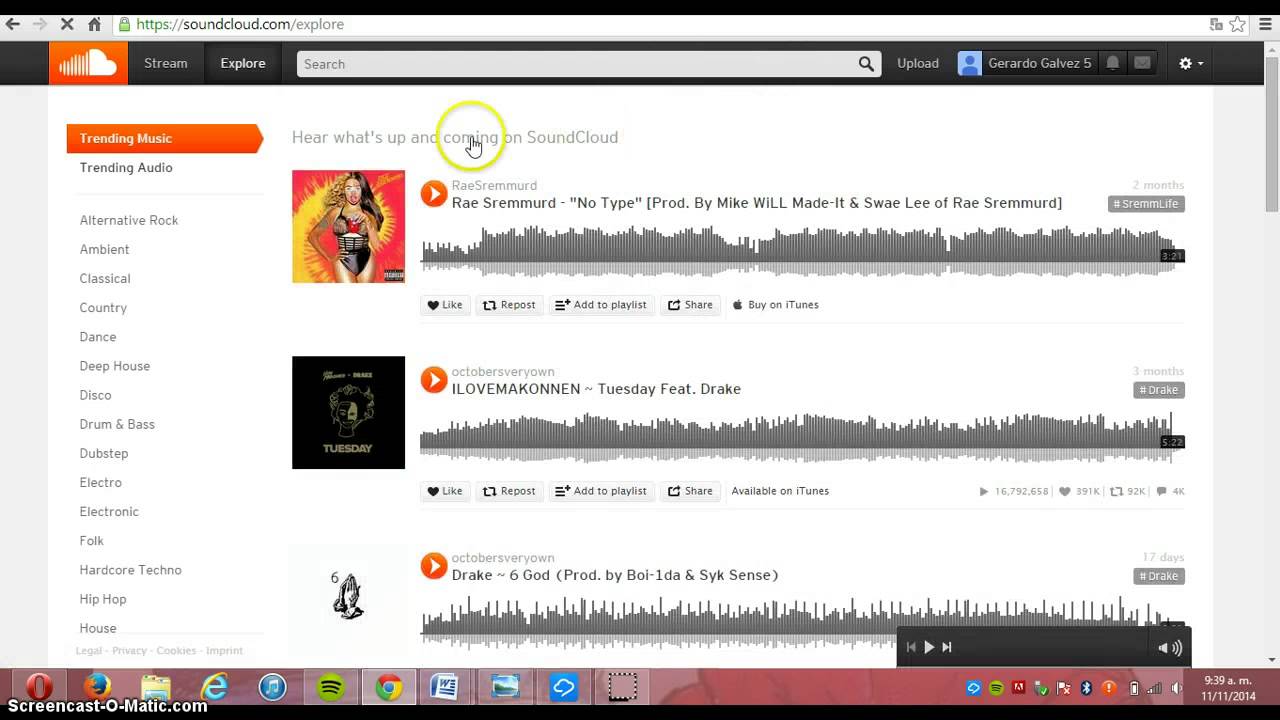The image captures the homepage of the SoundCloud website, specifically at the URL "https://soundcloud.com/explore," as shown in the address bar at the top. The iconic SoundCloud logo is prominently displayed, followed by the options "Stream" and "Explore." An empty search bar with the placeholder text "Search" and a magnifying glass icon to its right is located below. The "Upload" option is visible next to a profile icon and the name "Gerardo Galvez."

On the left-hand side of the page, "Trending Music" is highlighted in orange, followed by various music genre links including "Trending Audio," "Alternative Rock," "Ambient," "Classical," "Country," "Dance," "Deep House," "Disco," "Drum," "Dubstep," "Electro," "Electronic," "Folk," "Hardcore," "Techno," "Hip-Hop," and "House."

In the center of the page, a headline reads "Hear What's Up and Coming on SoundCloud," with the word "Coming" encircled in yellow and highlighted by a cursor. Beneath this headline is a thumbnail image of a woman with a play button, captioned "Rae Sremmurd - No Type (Produced by Mike WiLL Made-It and Swae Lee of Rae Sremmurd)." Below this is another thumbnail, featuring an image with a play button next to the title "ILoveMakonnen - Tuesday feat. Drake."